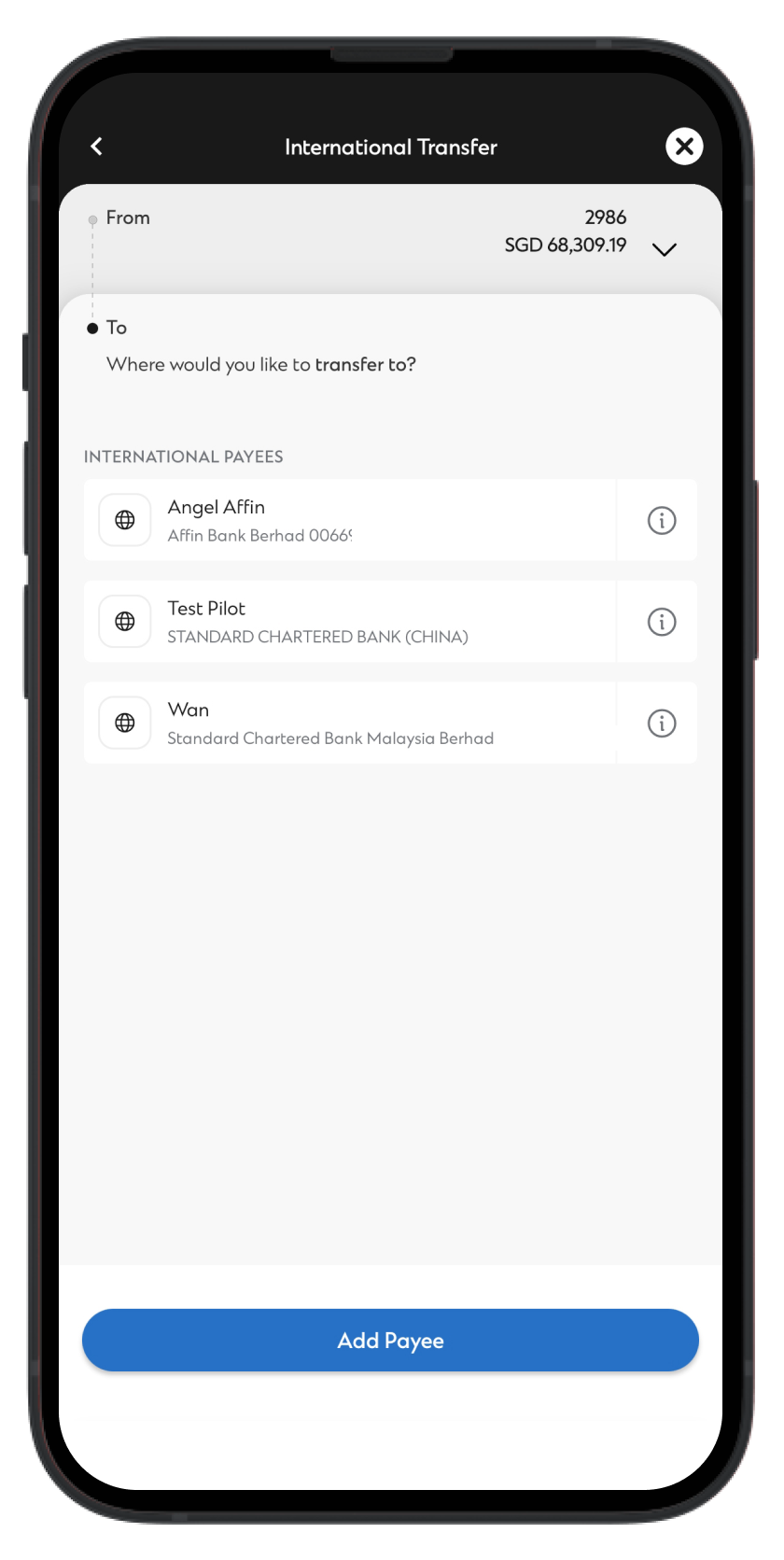Front and center, the image showcases a smartphone displaying an international money transfer page. The screen layout presents a clear depiction of financial activity:

- **Header Elements:**
    - An arrow on the left side to navigate back.
    - An "X" on the right corner to close the page.
    
- **Primary Details:**
    - The word "From" followed by the tab showing an amount of "2986". Directly beneath it, "SGD" is displayed.
    - Below this is an amount reading "680309.19" in a drop-down box.

- **Secondary Details:**
    - On top of the "From" section, lies another segment labeled "To".
    - The question "Where would you like to transfer to?" prompts user action.
    - This section lists:
        - **Angel Affin (Angel Bank Berhad)** with a reference "0.0066" and an information button labeled "Test Pilot".
        - **Standard Chartered Bank (China)** with an information button.
        - **Standard Chartered Bank (Malaysia)**.

- **Footer Elements:**
    - At the very bottom, the app offers an option to "Add Payee" in white text on a blue button.

- **Smartphone Features:**
    - The top part of the app screen is black.
    - Visible physical elements of the smartphone include:
        - Volume up and down buttons on the left side.
        - A slider button to mute them.
        - The power button protruding from the right side.

This detailed description encapsulates the image's content, focusing on the various interactive elements and the physical attributes of the smartphone.